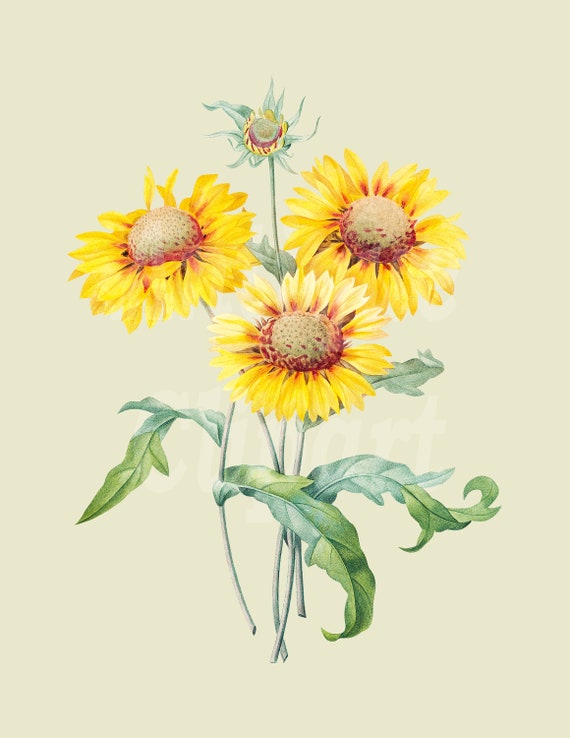This image showcases a detailed painting of sunflower plants on a cream-colored background with a light green frame. The central focus is on four sunflowers: three are fully grown, boasting vibrant yellow petals that encircle large tan-colored centers with reddish accents and smaller red and cream-colored buds. Their stems are a mix of greenish-blue and white hues, supporting the flowers and extending downwards. Each stem is adorned with two to three elongated, two-toned green leaves, featuring a unique blend of bluish-green and regular green shades. Additionally, there is one half-grown sunflower at the top, with wilted yellow petals and bluish-green remnants, adding a touch of realism to the artwork. The intricate details of the stems and leaves, coupled with the vivid depiction of the sunflowers, make this painting a captivating representation of natural beauty.